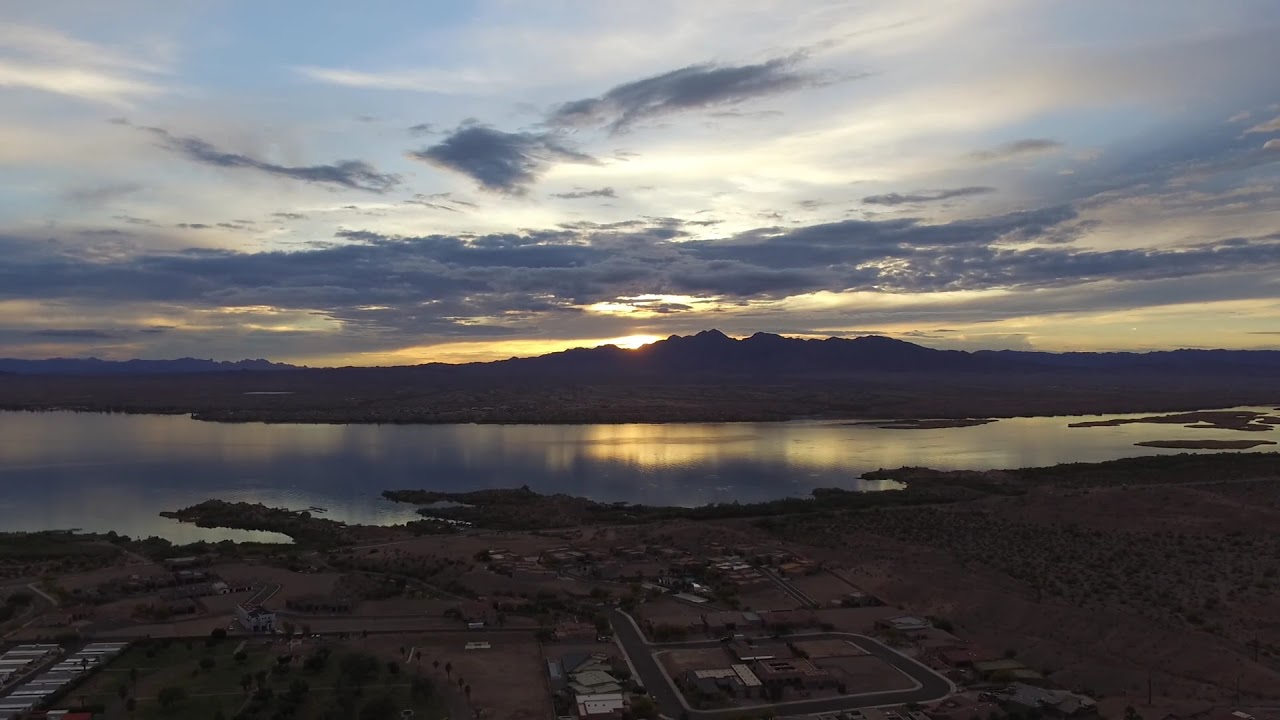The image captures an overhead, aerial view resembling the perspective from an airplane or drone, showcasing a sprawling landscape. Dominating the top half of the picture is a sky filled with a few clouds, one notably large. Below, a serene body of water reflects the vibrant hues of a sunset, which is the focal point and sets against a backdrop of distant mountains. The sun is partially obscured by the mountain range, casting a stunning array of colors that stand out against the otherwise drab and dark tone of the image. In the bottom left corner, neatly arranged, uniformly rectangular buildings or houses mark a small, secluded neighborhood. This area is interspersed with roads and vast patches of nature, including grass and dirt, reflecting a blend of community and wilderness. The picture vividly captures the balance between natural and human-made elements in a tranquil, somewhat isolated setting.